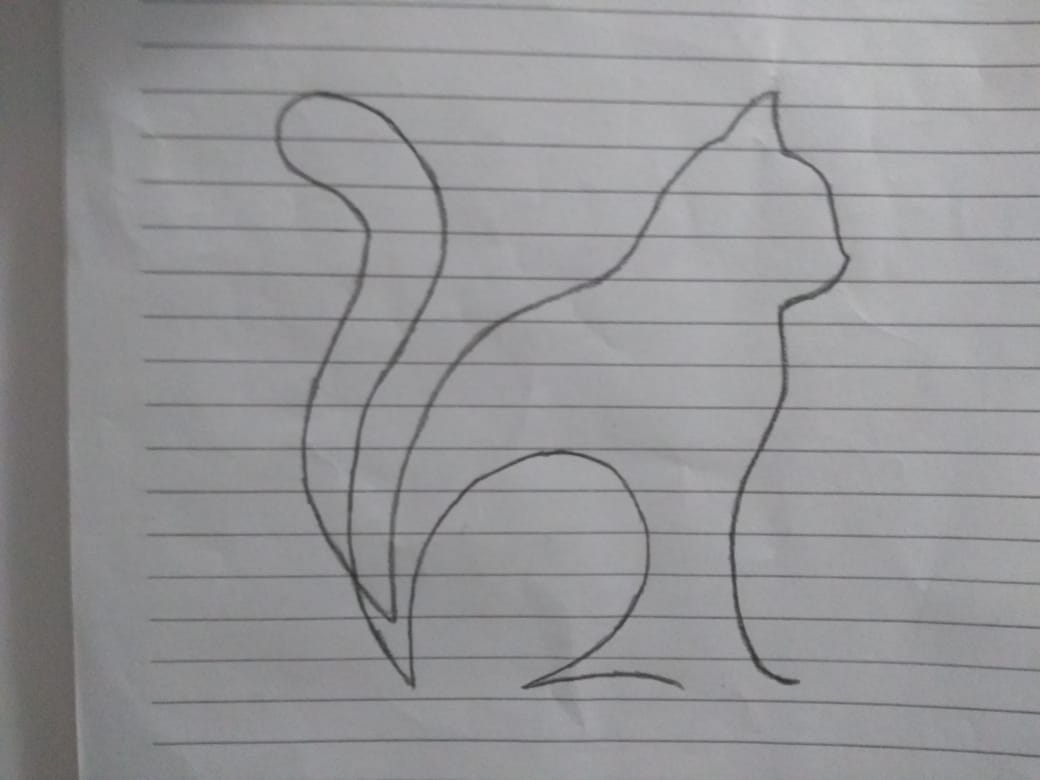A detailed line drawing depicts a cat sitting in a poised position, facing right in a side profile view. The outline captures the cat’s features intricately, from its pointed nose and ears to its strong hind legs and front paw extending forward. The artwork is rendered on a textured paper background, accentuated by multiple vertical lines that add depth and dimension. Notably, the cat's tail, which extends gracefully behind it, is whimsically illustrated as a large, wavy tongue, injecting a playful element to the otherwise elegant sketch.